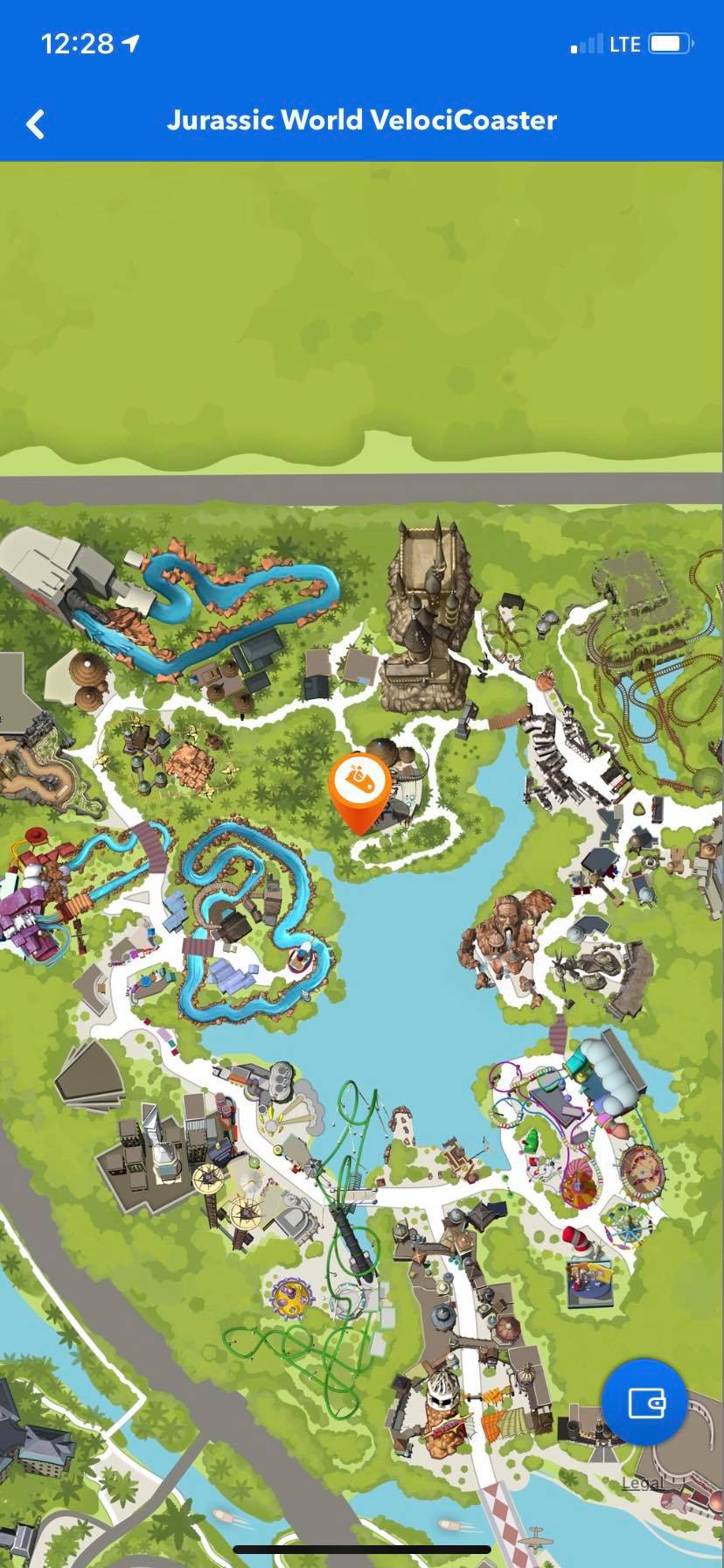The image is a smartphone screenshot featuring a watercolor-style top-down illustration. At the top, a bright sky-blue border frames the screen, displaying the time "12:28" in white font on the left. Opposite the time, in the top-right corner, icons for battery life and LTE signal strength are visible. Centered beneath the border, the headline "Jurassic World Velocicoaster" appears in white text.

The main portion of the image is a stylized watercolor map depicting the Jurassic World Velocicoaster area. The grass is rendered in varying shades of olive green, providing an earthy backdrop. Central to the illustration is an irregularly shaped, light blue body of water, somewhat reminiscent of a star's points. Several roads traverse the landscape, indicated by white and gray lines. Various landmarks and elements are outlined in shades of sky blue, adding a subtle depth and highlighting key features within the scene.